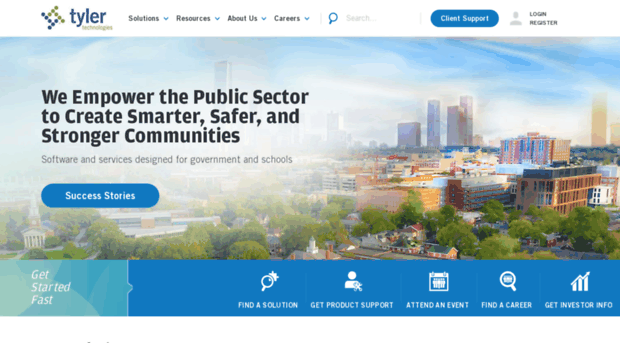The image features a white banner at the top with the word "tyler" in lowercase, bold blue lettering on the left. Directly below, "Technologies" is written in a green mossy color. To the left of the text, there is a square logo with overlapping lines; the left side of the square is blue and the right side is the same mossy light green.

Moving to the right within the banner, a navigation menu is displayed. The first option, "Solutions," has a blue arrow pointing downwards, indicating a drop-down menu. Next is "Resources," which also triggers a drop-down menu. This is followed by "About Us" and "Careers," each accompanied by a downward arrow as well. 

A thin dividing line separates the menu from a search area. The search icon is a blue magnifying glass, slightly tilted to the right. Next to it is an oval button with a dark blue background and white text that reads "Client Support." Lastly, there is a gray user silhouette next to the word "LOGIN" in small black capital letters.

Below the banner, the image showcases a city skyline with several corporate buildings, a cloudy sky, and some trees. On the left side, bold black text declares, "We empower the public sector to create smarter, safer, and stronger communities." Beneath this, in smaller, less bold gray text, it reads, "Software and Services designed for government and schools." At the bottom, there is another oval button with a blue background and white text that says "Success Stories."